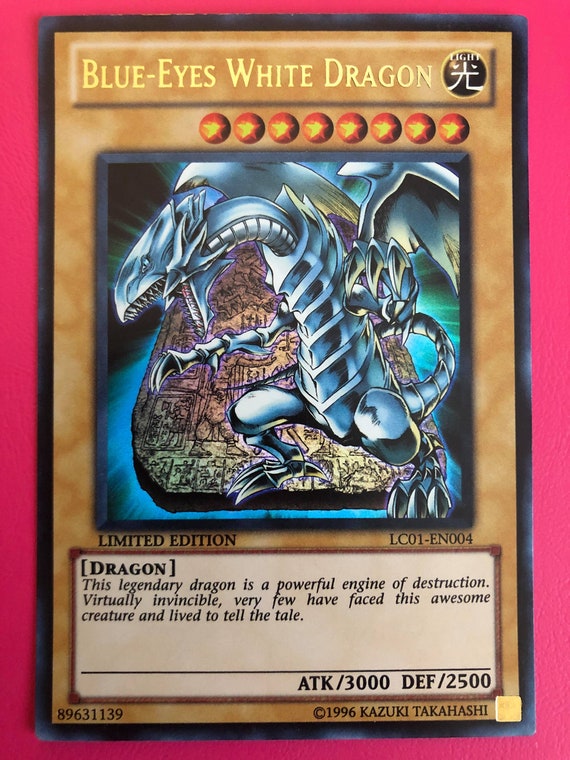This image is a detailed photograph of a Yu-Gi-Oh! card placed on a pink surface. The card features a distinct thin black border framing a marbled brown and white background. At the top, in prominent yellow text, it reads "Blue-Eyes White Dragon," accompanied by an Asian symbol in a circle. Directly below are eight red circles containing yellow stars serving as some form of rating.

The centerpiece of the card is a highly stylized depiction of a gigantic, silver, metallic dragon with a long neck, outstretched arms and legs, open jaws, and a downward-looking gaze. The dragon stands before a backdrop resembling an Egyptian-style tablet adorned with hieroglyphics. Below the image, "Limited Edition LC01-EN004" is inscribed, followed by a descriptor in a brown-bordered bracket stating "Dragon."

The card text reads: "This legendary dragon is a powerful engine of destruction. Virtually invincible, very few have faced this awesome creature and lived to tell the tale." Further down, a black bar separates this description from the combat statistics, listed as ATK/3000 and DEF/2500. At the very bottom, on the left side, there's a code "89631139," and on the right side, a small copyright notice reads "© 1996 Kazuki Takahashi."